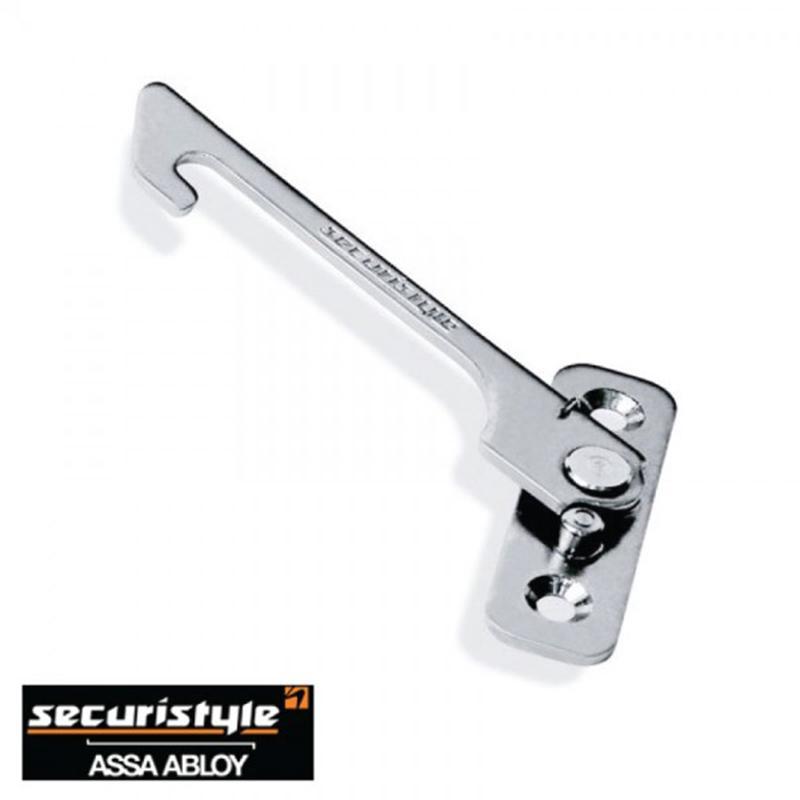This photograph features a silver tool, likely crafted from stainless steel or chrome-plated metal, identified as a window opening control device. The primary functionality of this device is to allow windows to open up to four inches for safety purposes, with an emergency release mechanism for further opening if necessary. It includes features such as a hook, swivel, mounting screw openings, a spring beneath, and an emergency button. In the image, the tool's branding is partially visible; it reads "Secura Style" in white print against a black background, along with the company name "Assa Abloy." Despite some blurriness rendering parts of the text unreadable, there is no mistaking the logo and branding. No other tools or persons are present in the photograph.